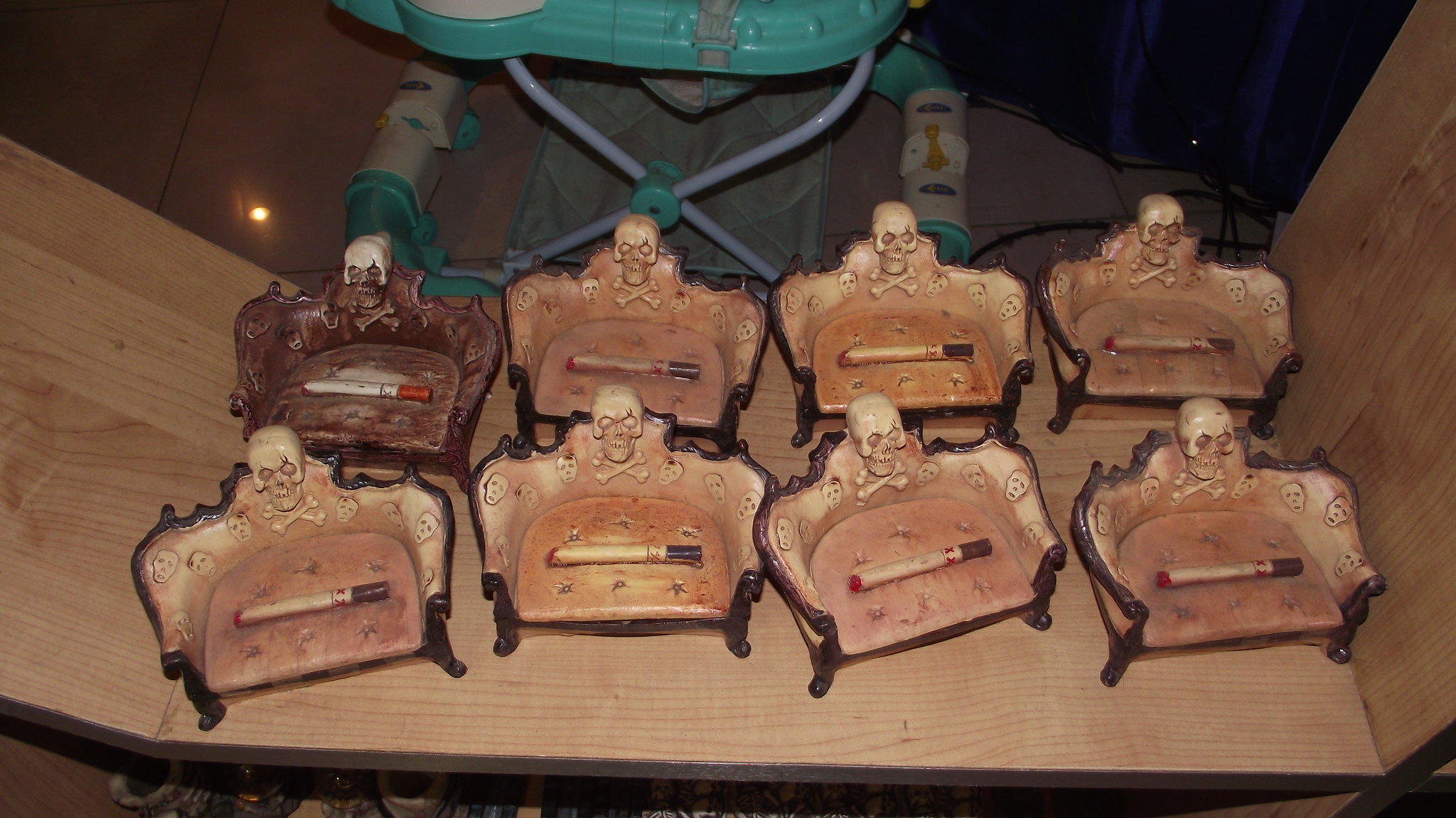This indoor color photograph prominently features a medium brown wooden shelf with sides, resembling a display case. Atop the shelf are eight identical, unusual doll-sized Victorian-style sofas, each featuring dark brown woodwork and antique distressed details. Each sofa's fabric is decorated with small skulls, with a larger skull carving and crossbones positioned at the back. There is a notable difference in fabric color: one sofa has dark brown fabric, while another combines cream-colored upholstery with skull designs. Perched lengthwise on the seat area of each sofa is an object resembling a lit cigarette, adding an eerie touch to the intricate miniatures. In the background, an aqua-colored baby walker with playful designs provides a sense of scale and hints at the photograph being taken in an attic or storage space.